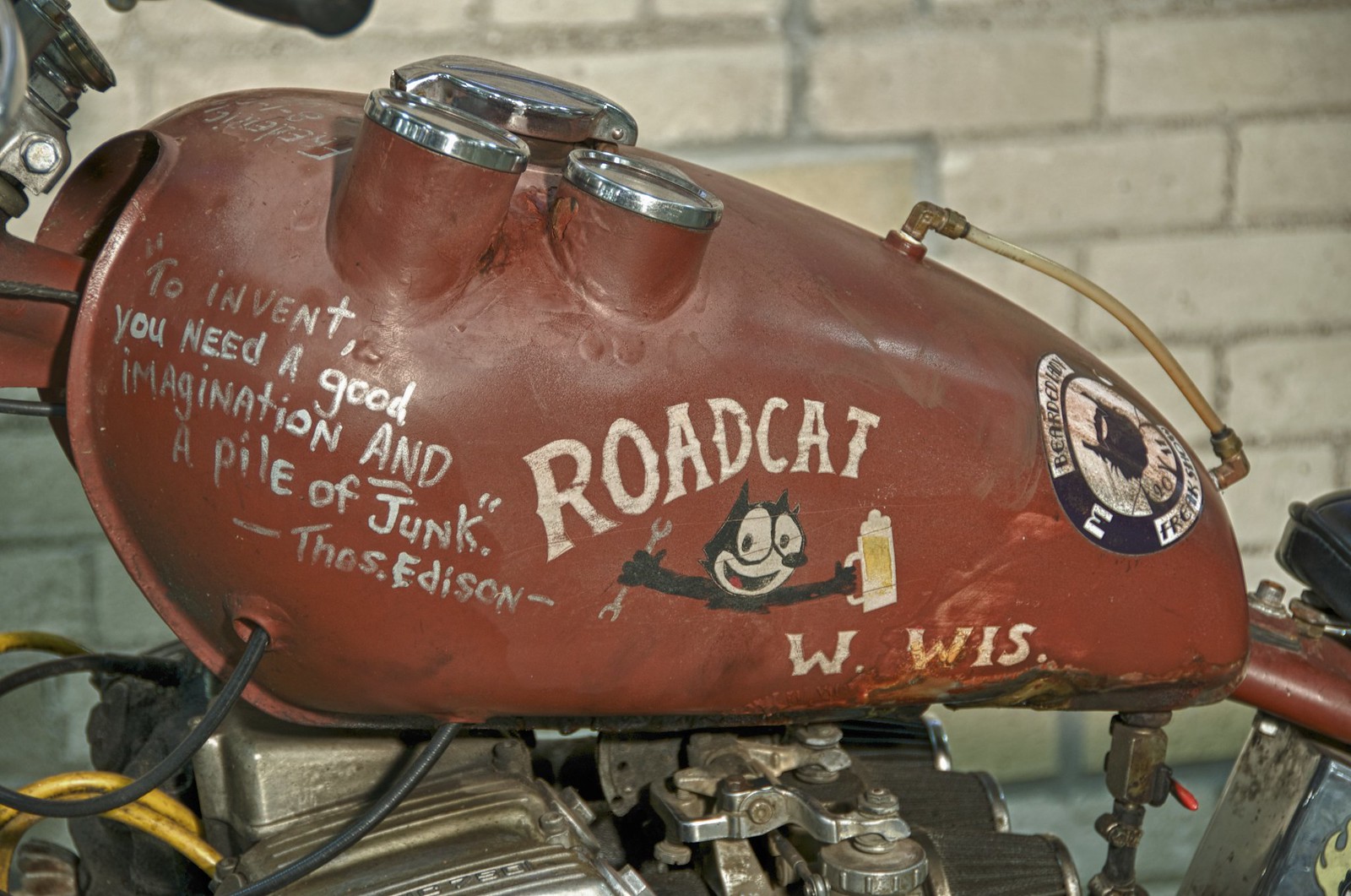This photograph depicts a vintage motorcycle, prominently featuring a rust-colored fuel tank adorned with a variety of detailed, nostalgic elements. The centerpiece of the tank is the logo "ROADCAD" etched in white letters, with an illustration of a black cat resembling Felix the Cat underneath. The cat, known as Bobcat, is distinctive with its white facial features, and it is cheerfully holding a wrench in one hand alongside a bottle, possibly glue or beer. Below the cat, the inscription "W.W.I.S." is visible.

On the left side of the tank, a famous quote is inscribed in silver: "To invent, you need a good imagination and a pile of junk," attributed to Thomas Edison, formatted humorously as "Toss Period Edison." The engine below the tank is entirely exposed, adding to the motorcycle's aged and rugged appearance. Additionally, other parts of the bike, like wires and components, are discernible, further emphasizing its vintage state. In the background, a brick wall adds to the rustic charm of the scene. This meticulously detailed fuel tank, likely from an early 20th-century motorcycle, serves as a testament to both the creativity and industrious spirit of the past.